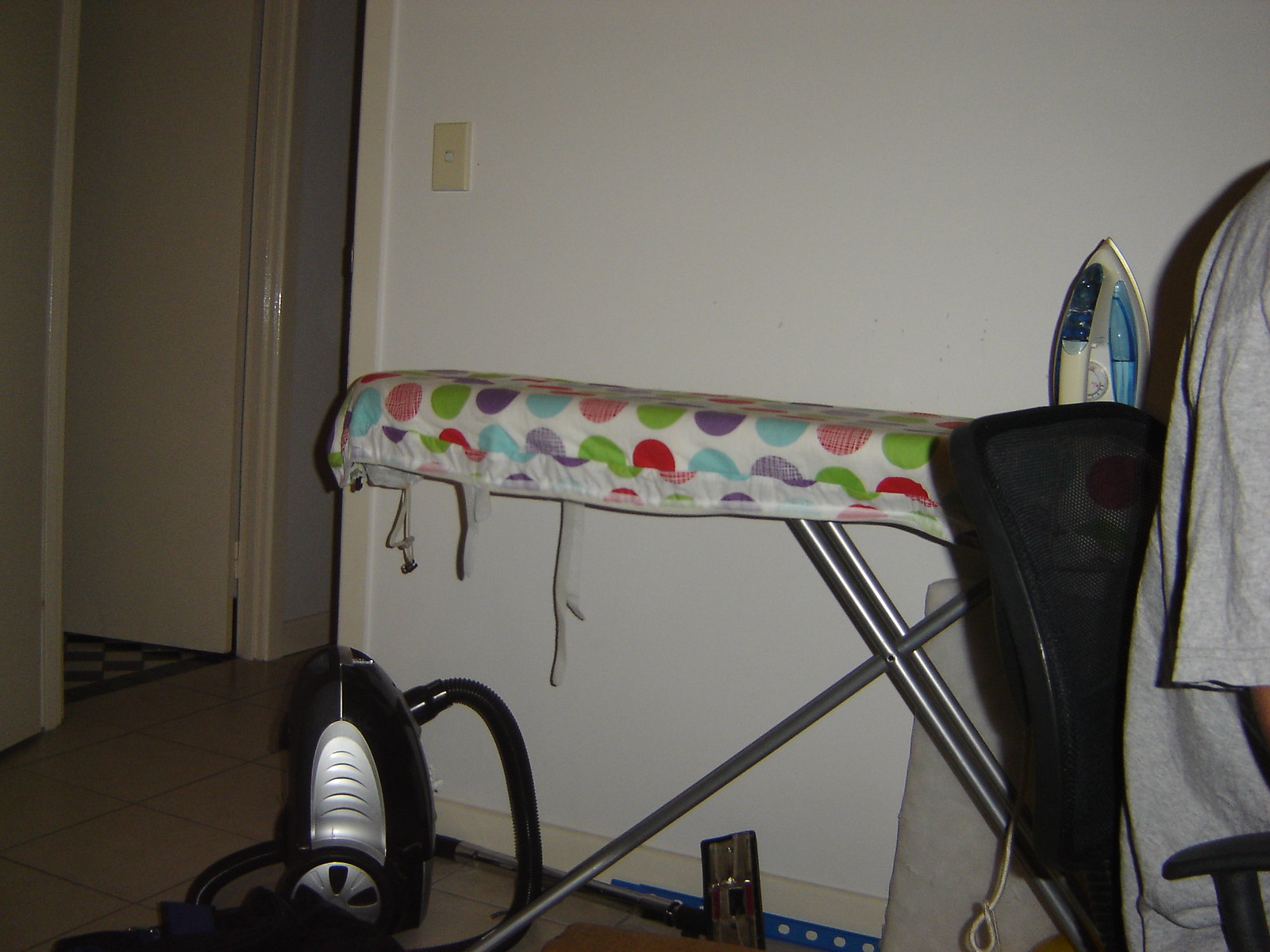This photo captures a room inside a home, the purpose of which is ambiguous—it could be a laundry room, utility room, living room, or even a bedroom. Dominating the scene is a plain white wall with an off-white trim. Against this wall stands an ironing board, covered in a unique fabric featuring multicolored polka dots arranged in a grid pattern—circles in red, green, purple, light blue, baby blue, pink, and lime green on a white background. At the narrow end of the ironing board sits an upright iron, white with a teal water chamber and a metallic rim.

On the floor to the left, underneath the ironing board, is a black canister-style vacuum cleaner with a silver panel and a long hose. Additional miscellaneous items, such as a Swiffer, hint that the room is used to store cleaning supplies. In the foreground, there's a black office chair occupied by a person wearing a gray t-shirt, with only their back and a bit of their shoulder visible. The floor is tiled, and there is an open doorway on the left, leading to another room with white walls and tiling.